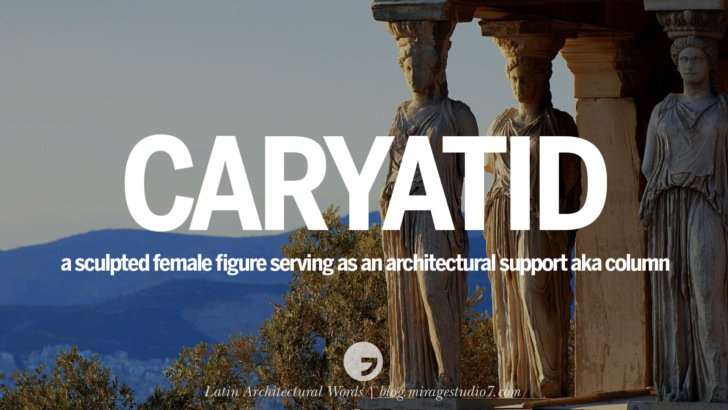The photograph captures an elegant scene of three statues of sculpted female figures, known as Caryatids, serving as architectural supports for a marble building. These figures, dressed in sleeveless white robes with low necklines, uphold large square-shaped carvings on their heads, which in turn support the roof above. Central to the image is white text that reads, "Caryatid, a sculpted female figure serving as an architectural support, aka column," further defining the statues' role. Smaller text at the bottom provides the source, "Latin Architectural Words, blog.miragestudio7.com." To the left, distant and grayish mountain ranges enhance the classical beauty of the scene, which is bathed in hues of gray, white, light blue, and green. The composition blends elements of natural landscape with classical architecture, creating a visually striking and informative piece that's evocative of ancient Roman or Italian temple structures.